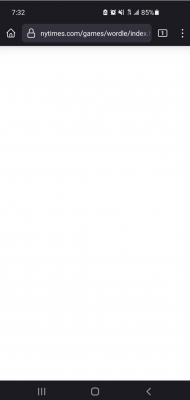A detailed caption for the described image could be:

"This screenshot from a smartphone depicts a blank webpage that has failed to load. Displayed at the top, the phone's menu bar shows the time as 7:32, with the battery saver active, an alarm set, and the device on vibrate mode. The phone has an 85% battery charge, indicated by a battery icon with a gray background. Below the menu bar, a search bar is visible with a truncated URL: 'nytimes.org/games/wordle/index...'. To its left, icons for a home button and a lock are shown, while to the right, a rectangular icon with a '1' indicates a single open browser tab. Further to the right, three vertically arranged dots signify the browser's menu options. The webpage itself is entirely blank, signifying it has either failed to load or is in the process of loading without displaying any content. At the bottom, the phone's navigation bar includes icons for recent apps, the home button, and the back button. The overall image portrays a straightforward and simple scene of a webpage loading issue."